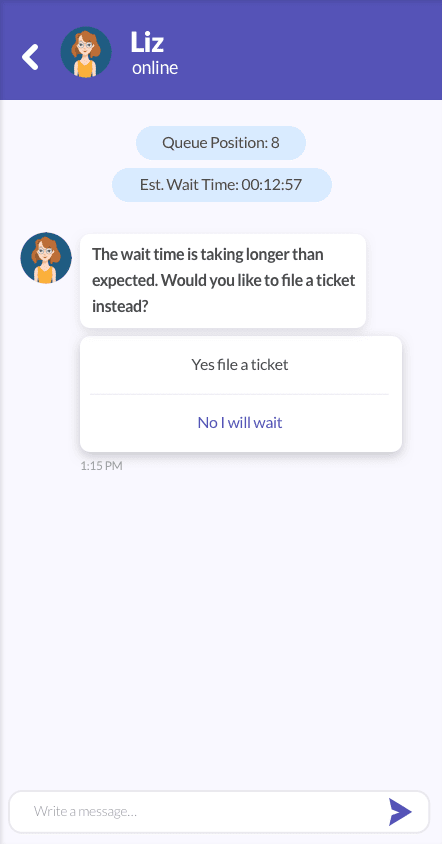A screenshot from a digital device, such as a phone, tablet, or computer, displays a chat interface where a user is conversing with an AI assistant named Liz. Liz's profile picture is a cartoonish avatar, suggesting she is an AI rather than a real person. The chat interface shows that the user is currently in queue position 8, with an estimated wait time of 12 minutes and 57 seconds. Beneath the queue information, there is a message from Liz, time-stamped at 1:15 p.m., informing the user that the wait time is longer than expected. Liz offers the user two options: to file a ticket by clicking "Yes, file a ticket," or to continue waiting by selecting "No, I will wait."